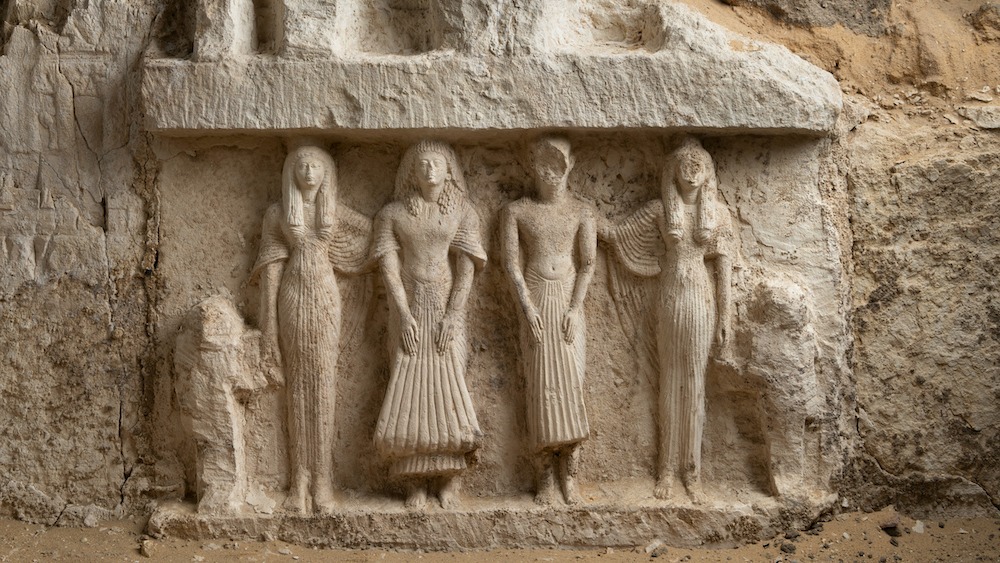The image captures a detailed carving on a light-colored stone wall, characterized by subtle shades of grey and brown, unearthed from the ancient Egyptian site at Saqqara. The relief features four adult figures arranged beneath a slight rock outcropping, reminiscent of a chapel or tomb entrance. Among the adults, three are women dressed in full-length gowns, with long hair cascading down their bodies, styled in the traditional ancient Egyptian manner. The fourth figure is a man, distinguished by a chipped face and clad in a white skirt. Flanking these adults are partially finished carvings of children, one on each side, indicating incomplete work on the stone. The overall scene exudes the historic aura of ancient Egypt, reflecting familial representations often depicted in Egyptian art, with intricate detailing emphasizing its antiquity and cultural significance.